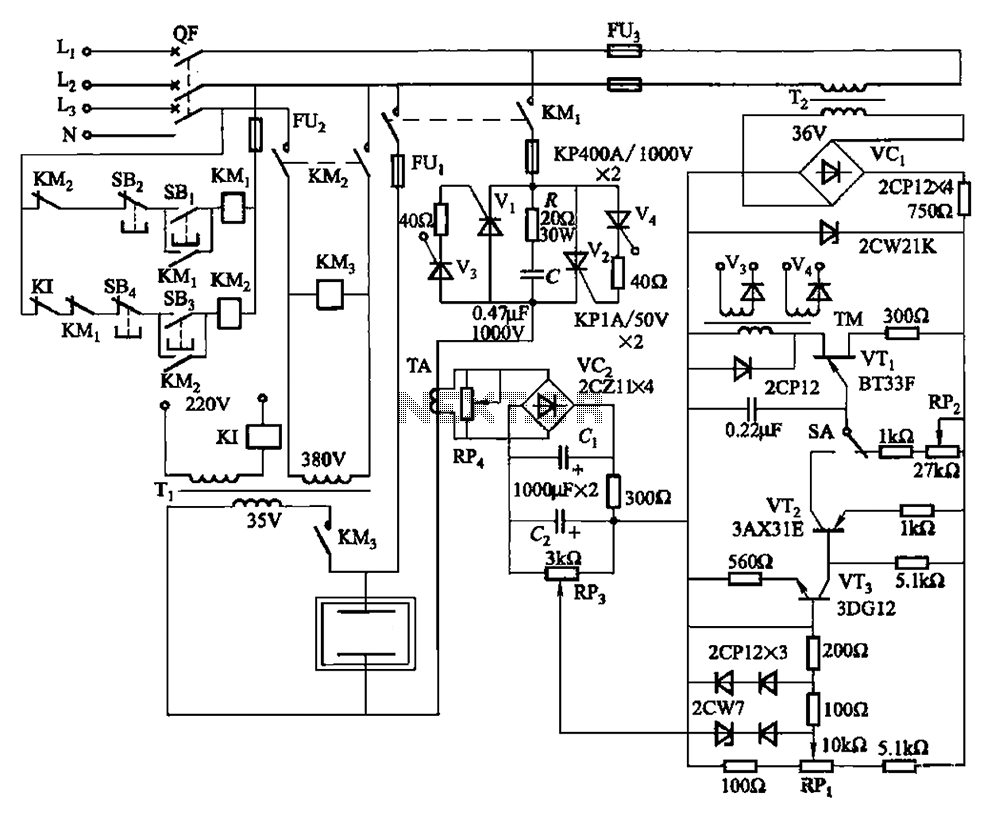The image is a highly detailed black and white digital line drawing of a complex electrical diagram set against a white background. At the center of the diagram are the prominently displayed words "Nexter" or "N-E-X-T-E-R". The diagram features numerous labeled components, including squares, diamonds, triangles, and a variety of intersecting lines. Key labels include "KM2," "KM3," "FU2," "380V," "L1," "L2," "L3," "N," and "KP400A/1000V". There are zigzag patterns, small black dots forming lines and words, and an array of interconnected circuits, resistors, and rectangular boxes. Despite its complexity and static nature, the diagram is indicative of an intricate electrical or engineering schematic, possibly meant for those with expertise in mechanical or electrical fields.